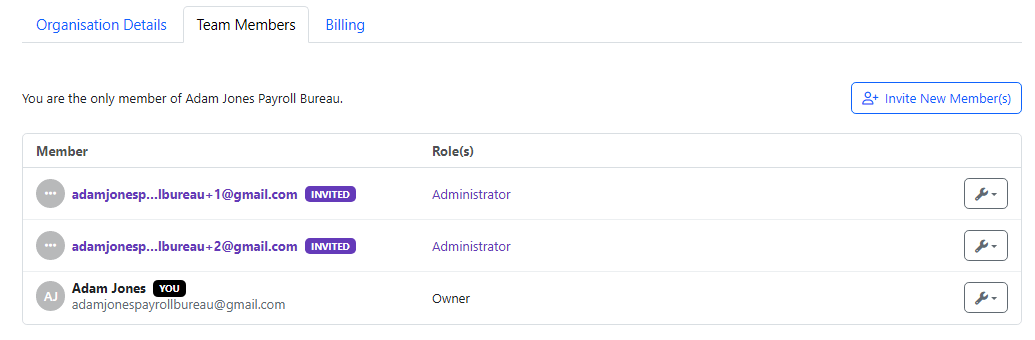Here is the refined and detailed caption:

---

The interface displays a predominantly white main page with blue text, and navigation tabs positioned at the top of the image. On the top left, the tabs read "Organization Details," "Team Members," and "Billing." "Organization Details" and "Billing" are written in blue to indicate they are not selected, while "Team Members," positioned between the two, is in black to indicate it is the currently active tab.

Below this top navigation, centered on the page, the text reads, "You are the only member of Adam Jones Payroll." To the right, there is an outlined button in blue with blue text that reads, "Invite New Members."

On the left side of the page, there is a table sectioned into two columns labeled "Member" and "Role." The table comprises three rows:

1. The first row contains:
   - Member: "Adam Jones Payroll Bureau plus one, sgmail.com"
   - Role: "Invited, Administrate" (in purple text)
   - A settings icon on the far right.

2. The second row contains:
   - Member: "Adam Jones Payroll Bureau plus two, sgmail.com"
   - Role: "Invited, Administrate" (also in purple text)
   - A settings icon on the far right.

3. The third row contains:
   - Member: "Adam Jones U, Adam Jones Payroll Bureau, sgmail.com"
   - Role: "Owner" (in black text).

These rows indicate the members associated with "Adam Jones Payroll Bureau" and their corresponding roles, highlighted by the functional settings icons at the far right of each row.

---

This caption provides a detailed and organized description of the interface elements and layout.